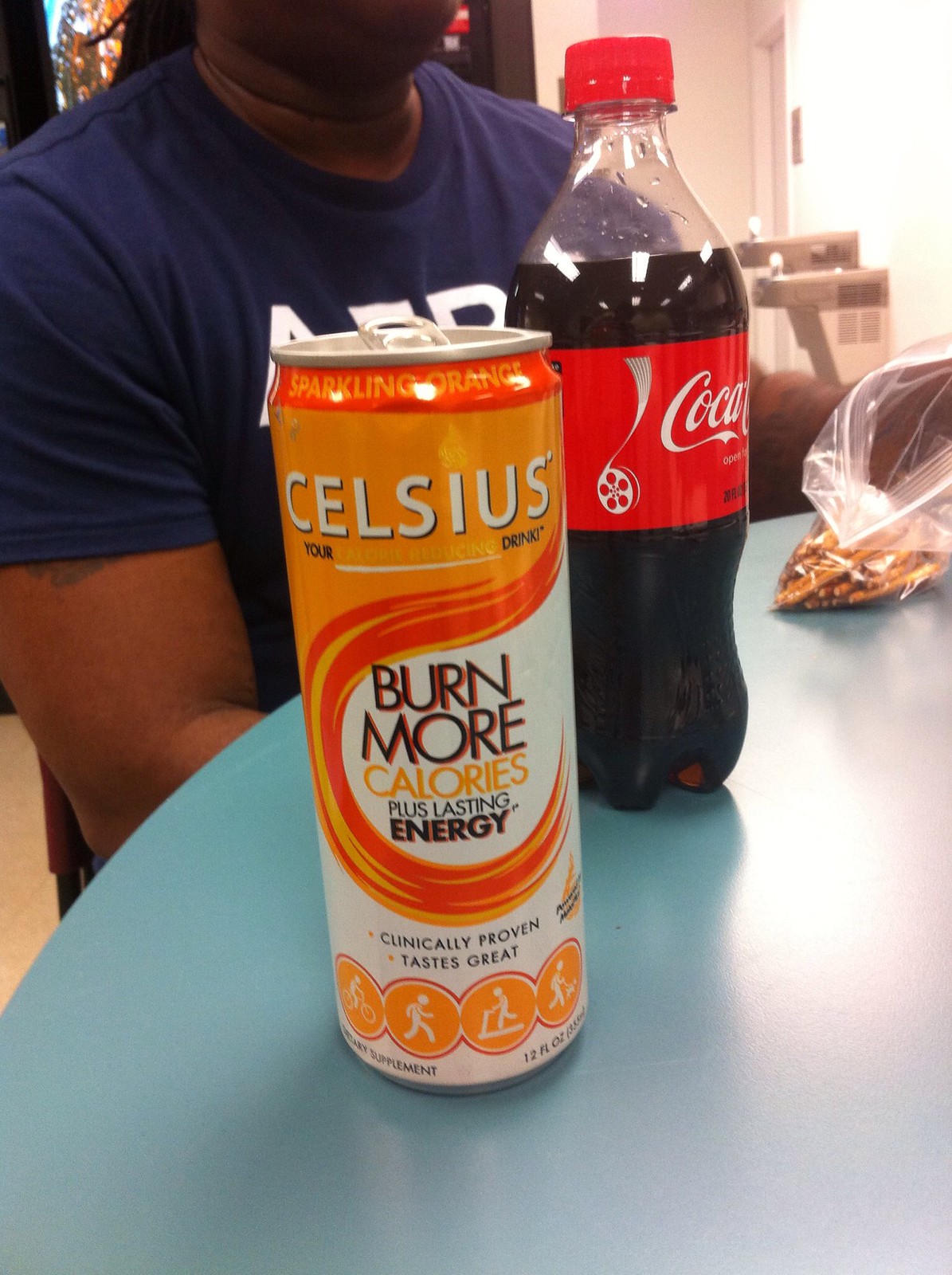In this detailed photograph, an African American man, muscular and tattooed, is seated at a light cyan blue circular table. His face is partially cut off in the picture, revealing only his chin down to his elbows, and he is wearing a short-sleeved dark blue t-shirt with visible tattoos on his forearm and upper arm. On the table, slightly in front of him, is a nearly full bottle of Coca-Cola, held in a clear plastic bottle with a distinctive red label and a matching red cap. The label also features a white movie reel motif. Next to the bottle is an orange and white cylindrical can of Celsius, which prominently displays the text "Celsius" in white. The can features a flame-like orange swirl design and claims to "burn more calories plus lasting energy." Additional details on the can include orange circular icons depicting a person biking, running, using a treadmill, and walking a dog. To the right of the can is a clear Ziploc bag containing pretzels. In the background, there's a white wall, a vending machine, and two white and gray rectangular objects whose purpose is unclear.